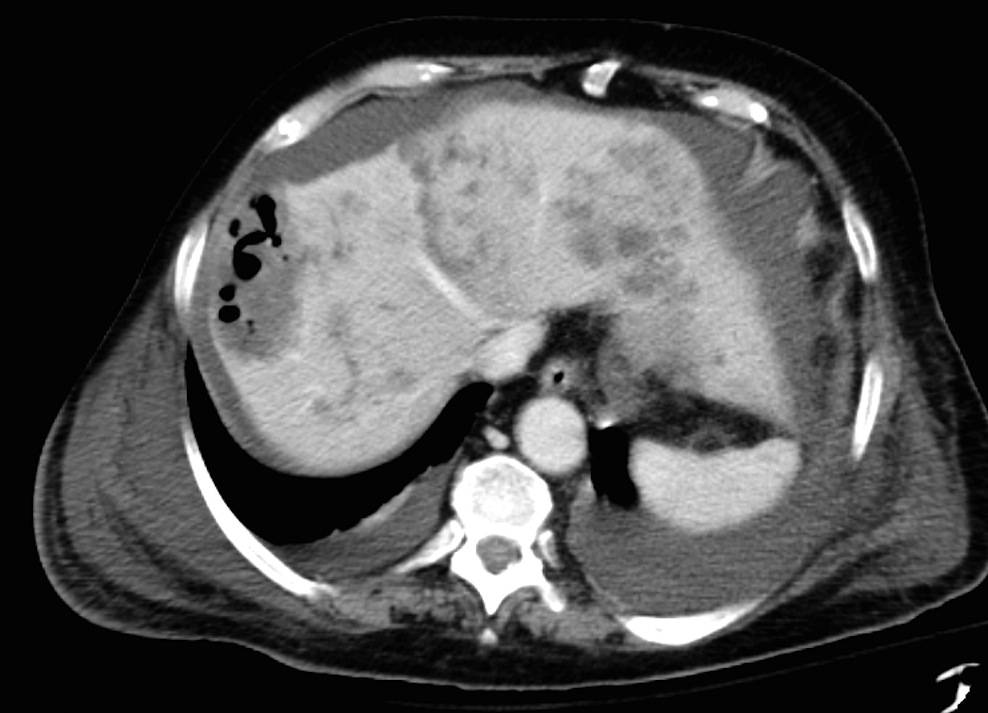The image is a black and white MRI scan of a human brain, displaying intricate details of its structure. The brain, which has a trapezoidal appearance, showcases various shades of grey. The middle region of the brain appears in a light grey tone, while the borders are darker grey. White streaks are visible in the organ, particularly around the borders and at the bottom middle. Noticeably, the bottom left side features a curved black portion that stands out against the lighter surrounding. The remainder of the background is uniformly black, enhancing the contrast and detail within the brain's image.